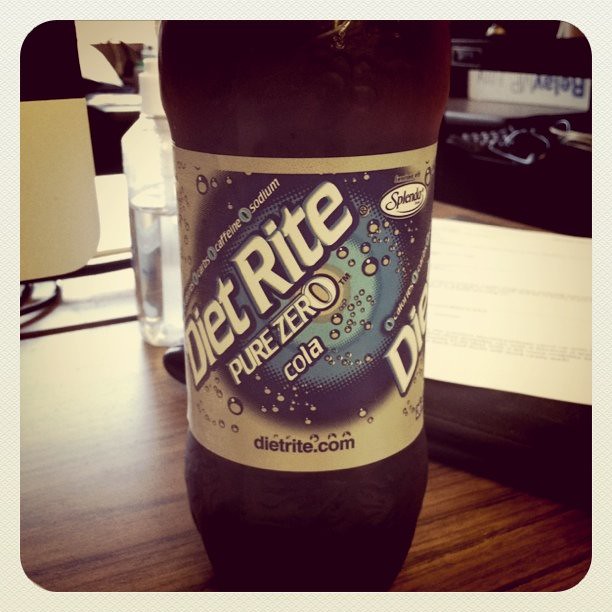The image features a bottle of Diet Rite Pure Zero Cola, prominently centered to showcase its label. The label design is distinguished by a white-to-light-blue gradient, with dark blue rings at the edges that transition to a lighter blue and finally to white at the very center. The logo and name "Diet Rite Pure Zero" are printed in white against this background. Notably, the website "dietrite.com" is listed at the bottom of the label. The bottle, clearly filled with the cola, reveals the dark, characteristic color of the beverage through sections at the top and bottom. The entire setup rests on what appears to be a standard table.